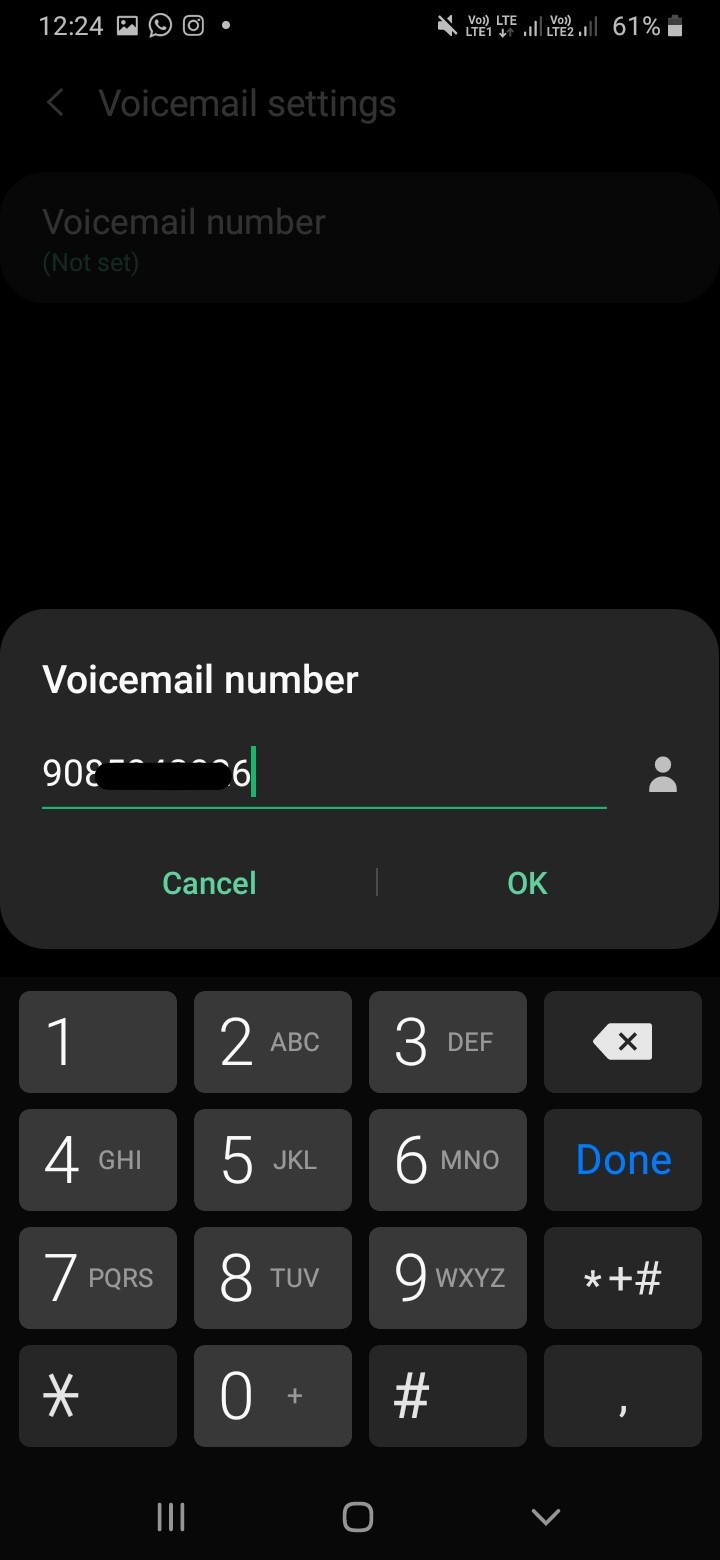The image depicts a user's cell phone screen displaying a voicemail settings interface with a predominantly black background. At the top left corner, the time is shown as 12:24 PM in white text. Adjacent to this are various status icons, including voicemail, photos, and a notification indicating that notifications are turned off. The battery icon, showing a 61% charge, is located on the far right.

The main portion of the screen is dominated by the voicemail settings. "Voicemail Settings" is written at the top in a pale gray color, accompanied by a back arrow icon. Directly beneath it is the heading "Voicemail Number." The screen features a lighter black, horizontal rectangular box with "Voicemail Number" labeled in white text at the top. Inside this box, a white voicemail number is partially obscured with black markings for privacy.

Further down, there are two actionable options displayed in green text: "Cancel" and "OK." Below these buttons is a numeric keyboard layout, presented in several horizontal rows. The layout includes:
- Row 1: Number keys 1, 2, 3, followed by a delete (X) button.
- Row 2: Number keys 4, 5, 6, followed by a bright blue "Done" button.
- Row 3: Number keys 7, 8, 9, with a combined asterisk (*), plus (+), and pound (#) key.
- Row 4: Keys for asterisk (*), 0, and pound (#).

At the very bottom of the screen, there are three navigation icons: three horizontal lines representing the menu, a home icon for the home page, and an additional down arrow for further options.